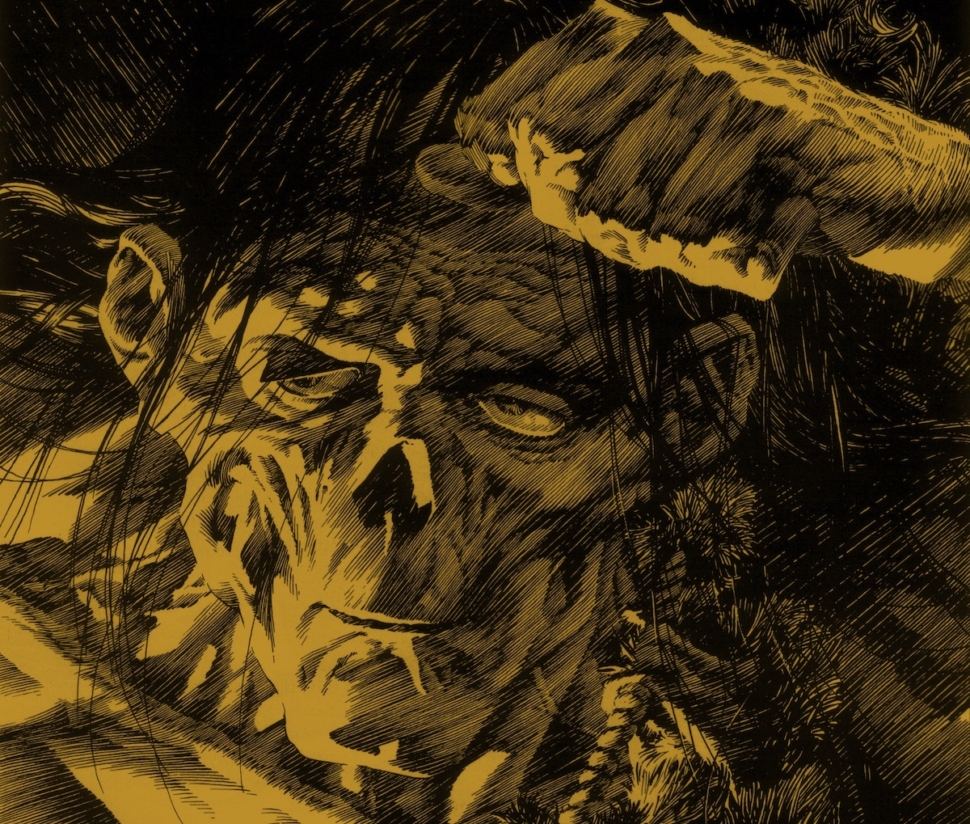The image is a detailed, pencil-drawn or painted depiction of a skeletal, prehistoric caveman-like figure with a haunting, emaciated appearance. It's suffused in hues of yellow, gold, black, and gray, with no traces of white. The caveman's head, centered and dominating the middle of the composition, showcases a sunken-in face, skeletal features, and missing nose revealing the nasal cavity. Dark, thin, long hair cascades from the top middle, above his wrinkled and almost brain-like brow. A clenched fist rises above the head on the far right, with the forearm leading down. Below the fist, in the bottom right corner, some flowers are visible. The composition has a sci-fi or comic-like aesthetic, with the left side of the face highlighted by a light source, enhancing the eerie skeletal visage, and the overall atmosphere hinting at the caveman's formidable yet deathly presence.